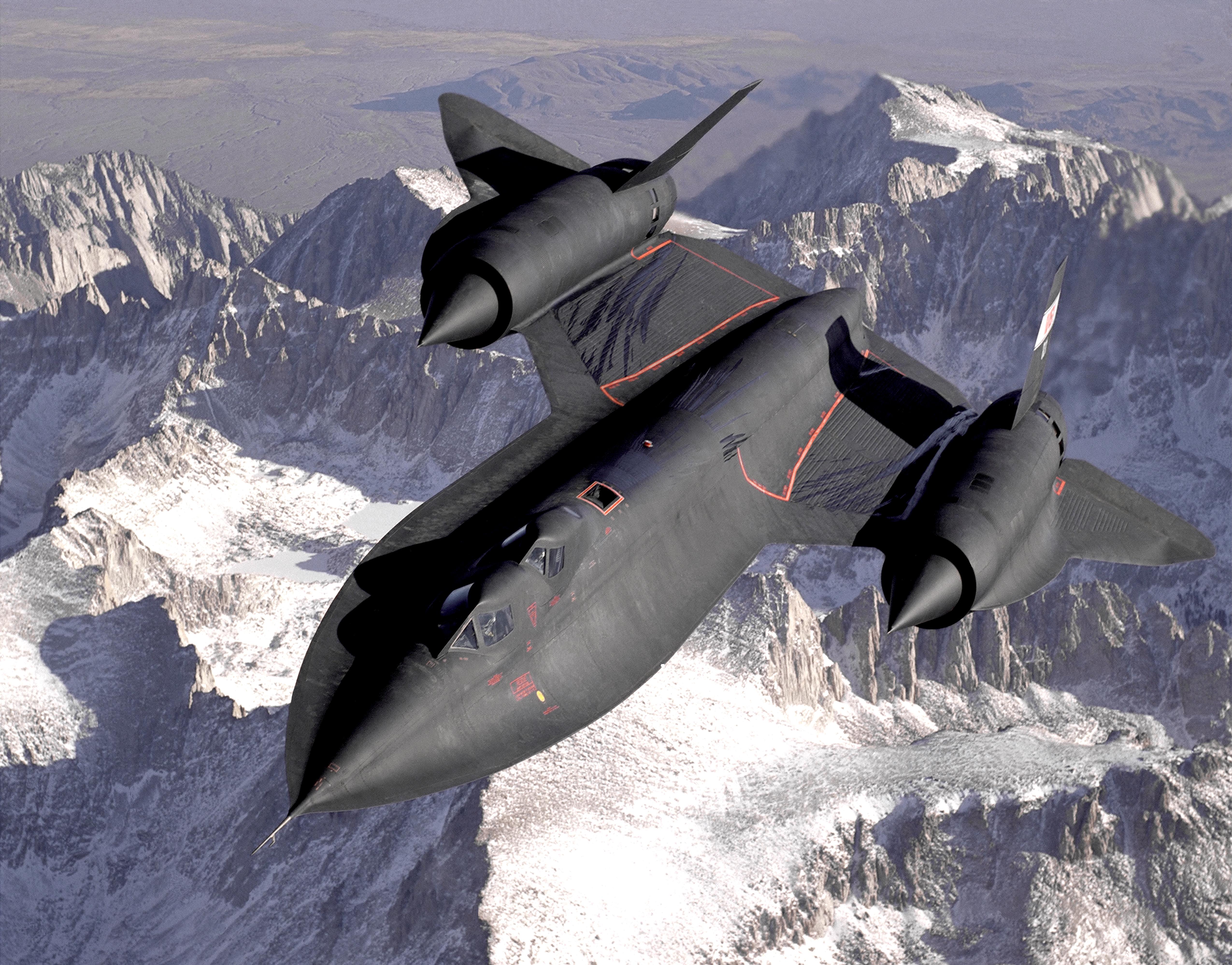A striking image captures a sleek, all-black stealth fighter jet soaring over a majestic mountain range. The jagged, steep peaks below are blanketed in pristine snow, creating a dramatic contrast with the dark aircraft. The jet features a streamlined design with two level wings extending from its rear, each housing one of the two powerful engines. These engines are notable for their sharp, cylindrical intakes at the front and fins at the rear, enhancing the plane's aerodynamic profile. The aircraft's body widens slightly along the sides before tapering into a sharp nose, accented by a silver rod at the front.

Centrally positioned on the jet's fuselage are two sets of windows. The raised compartment towards the middle hosts triangular windows, while a line of square windows is situated to the right, one behind the other, giving the aircraft a futuristic and efficient appearance. The overall design exudes an aura of cutting-edge technology and stealth capability, set against the breathtaking backdrop of snow-capped peaks.